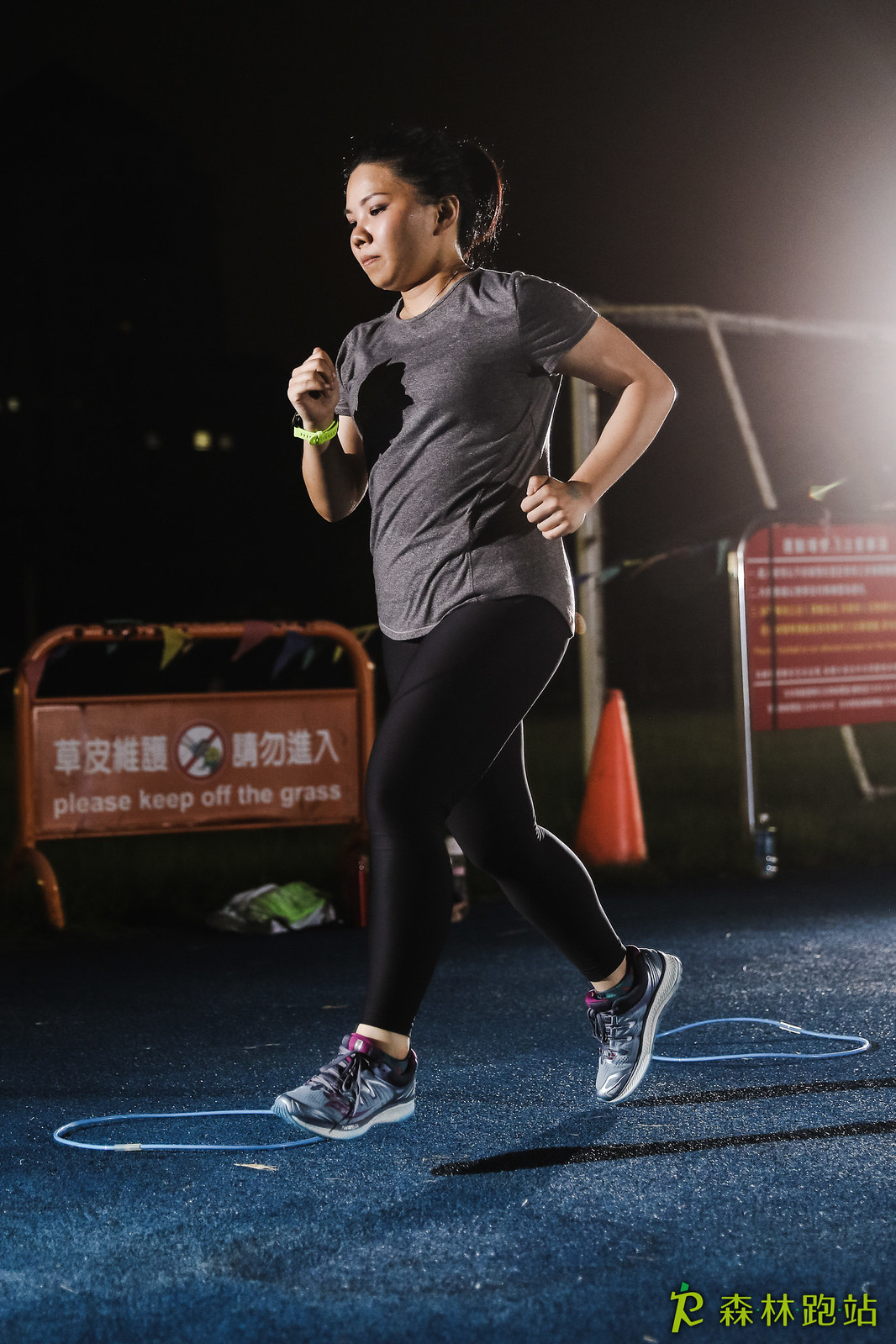The nighttime scene captures a woman of Asian descent mid-jog, with her gaze focused downward, running across a black concrete surface accented by small circular blue objects. She is wearing a short-sleeved gray shirt, long black leggings, black sneakers, and a green wristband on her right wrist. Her black hair is tied back, and she has olive-colored skin. Behind her, partially visible, is an orange traffic cone, a barrier displaying the words "please keep off the grass," and a red sign with white and yellow text. To her side, there's a soccer goal, and in the lower right-hand corner of the image, lime green characters in either Chinese or Japanese script can be seen. The background is pitch black, emphasizing the nighttime setting.